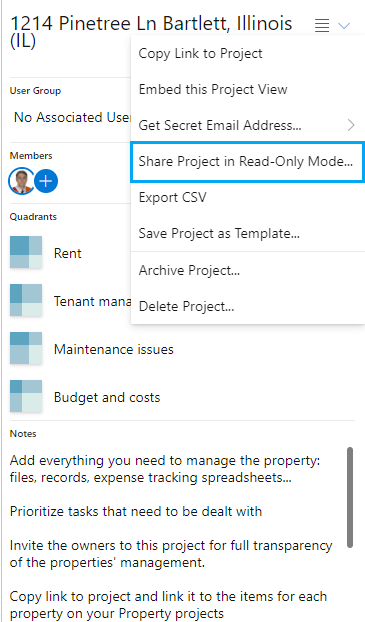The color image appears to be a screenshot taken from a digital device, likely a cell phone or computer monitor. The image is rectangular, with the longer side oriented vertically. 

The primary background color is white, and it features black text prominently. At the top, in larger, bold black letters, it displays the address: **"1214 Pine Tree Lane, Bartlett, Illinois."**

Below this address, there is a functional menu with a series of options presented in a dropdown bubble format:
1. **Copy Link to Project**
2. **Embed This Project View**
3. **Get Secret Email Address**
4. **Share Project in Read-Only Mode** (highlighted with a light blue square indicating it is selected)
5. **Export CSV**
6. **Save Project as Template**
7. **Archive Project**
8. **Delete Project**

At the bottom of the dropdown menu, there is additional descriptive text:
- **Notes:** "Add everything you need to manage the property. Files, records, expense tracking spreadsheets."
- **Prioritize tasks that need to be dealt with.**
- **Invite the owners to this project for full transparency of the project's management.**
- **Copy link to project and link it to the items for each property on your property projects.**

This detailed menu seems to be part of a property management application or platform, designed to facilitate various aspects of property administration and collaboration.